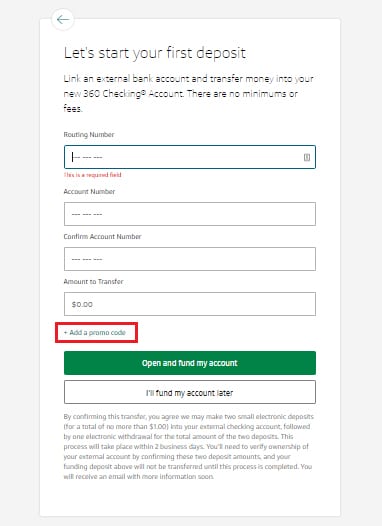The screenshot displays a user interface for initiating a first deposit into a new 360 Checking account. At the top, a prominent header reads, "Let's start your first deposit." Directly below it, instructions guide the user to link an external bank account and transfer money, highlighting that there are no minimums or fees involved.

The main section features four input fields aligned vertically:

1. The first field, highlighted in green, is labeled "Routing Number."
2. The second field is labeled "Account Number."
3. The third field is labeled "Confirm Account Number."
4. The fourth field is marked "Amount to Transfer," currently set to $0.00.

While the Routing Number field is highlighted, the other three fields are in a gray tone.

Below these fields, there's a red rectangle containing the phrase "Add a promo code" in light blue text. Further down, a green rectangle with white text reads "Open and fund my account." Beneath this is a white rectangle with black text stating, "Fund my account later."

At the very bottom of the screen, there is a small paragraph of light gray text. The entire page has a white background, bordered by a light gray background on the left, right, and top edges.